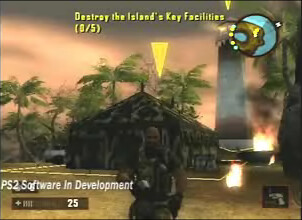This is a low-resolution screen capture from a military-style shooter video game, resembling early development or alpha stage for the PS2, as indicated by the white watermark reading "PS2 software in development" in the corner. The image's bottom edge shows the player's gun, a black object pointed forward, while the health is displayed at 25 in the bottom left corner. The top right corner features a mini-map with the player's position as an arrow among various objective-representing dots. At the top of the screen, an objective caption reads, "Destroy the island's key facilities, 0 out of 5," with a prominent yellow arrow pointing toward a small dark, possibly wooden shack-style building amidst tropical palm trees and a lighthouse in the distance. The central character, who vaguely resembles Rambo in a body armor vest, is mostly blurry, adding to the scene's overall low-res appearance. The background includes a camouflaged barracks or tent, palm trees, and an obelisk similar to the Washington Monument with visible fire near its base, adding to the setting's tension and urgency.